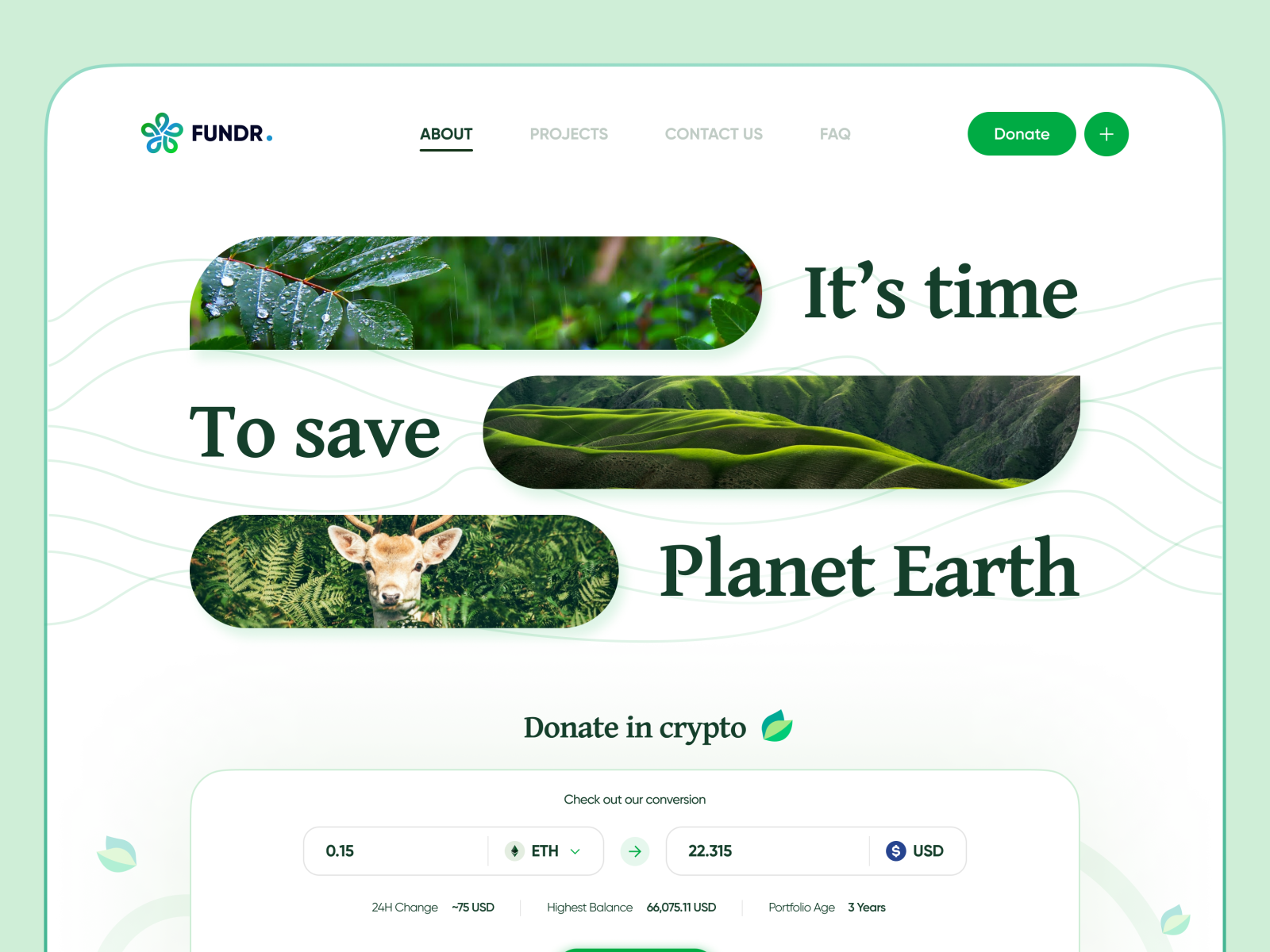This image is a screenshot of a website called "Funder," which appears to be dedicated to environmental conservation. The layout features a green border with a slightly lighter green outline and a large white central section. The bottom part of the image is cut off, so the border is not visible there. 

At the top of the image, there is a green and blue logo next to the text "Fund R." Following this, in the center-top area, there are four navigation buttons. The "About" button is highlighted in dark green. Next to it are "Projects," "Contact Us," and "FAQ," all in grey text. On the far right, there is a bold green button with white text that reads "Donate," and next to it, a green circular button with a white plus sign.

In the middle section of the image, three nature-themed shapes contain images of leaves, hills, and a deer in a forest. Bold green text beneath each image states, "It's time to save planet Earth." Below this, in smaller font, is the text "Donate in Crypto" accompanied by a leaf icon.

At the bottom is an image displaying a cryptocurrency transaction page with a white background, specifically indicating an exchange from Ethereum to USD.